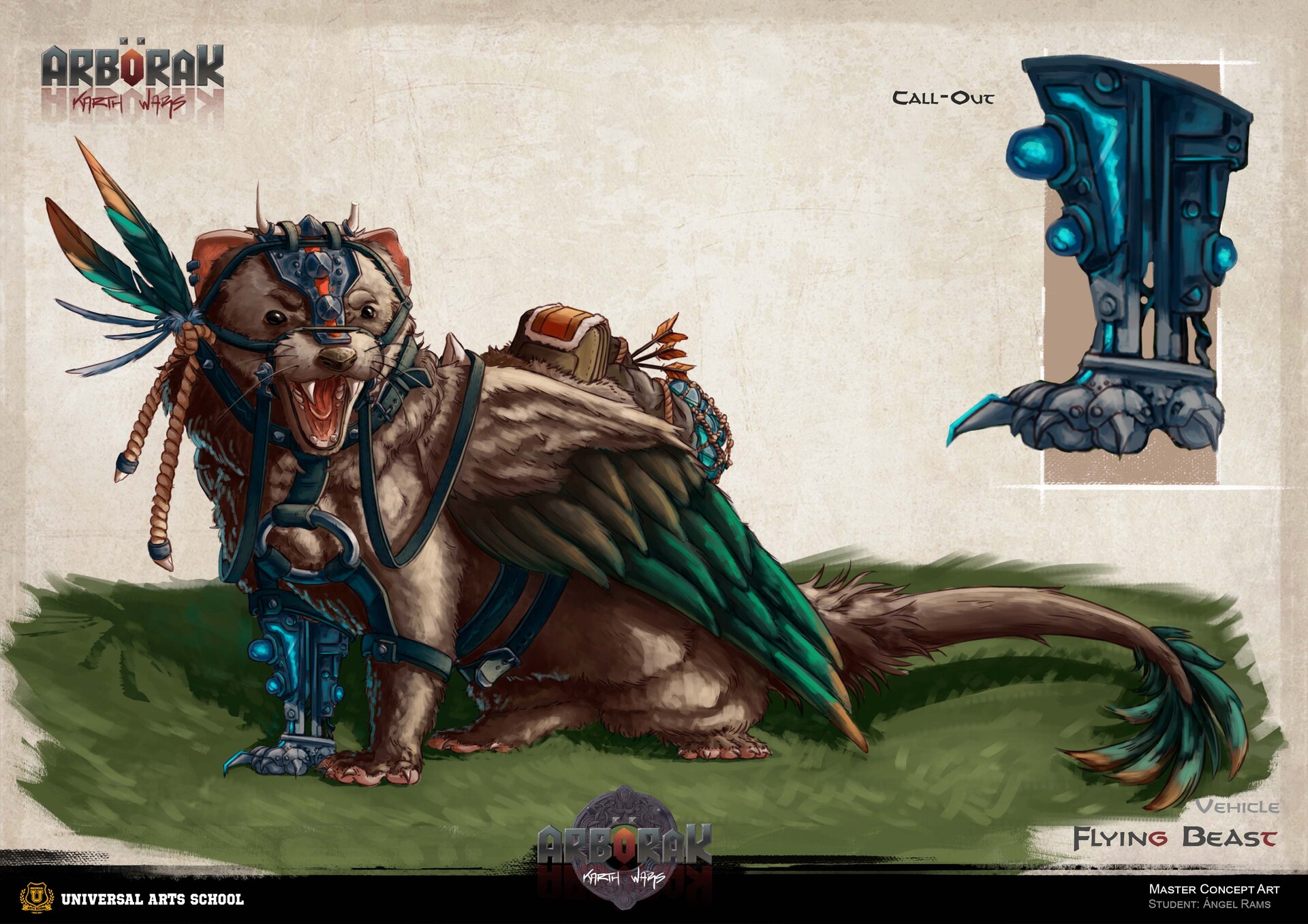This detailed rendering titled "Arborac" from the Universal Arts School, created by Master Concept Art student Angel Ram, showcases a fantastical, possum-like flying beast. The creature, central to the design, is depicted with a fusion of avian and rodent features—its body boasts a striking array of alternating green, gold, tan, maroon, red, gray, and black feathers. The beast's large, incisive teeth are exposed as its mouth opens, and its muzzle, decorated with peacock feathers and a braided rope cord, adds an exotic touch. Its long tail, adorned with peacock-like feathers at the end, aligns with the intricate, claw-like armor on its chest. Notably, its paws are detailed with claws, one of which is highlighted in a call-out in the upper right. The art piece includes text at the bottom proclaiming the creature as the "Vehicle Flying Beast," with the term "Arborac" and the Universal Arts School's logo also prominently displayed. A mysterious blue and gray object sits to the side, adding an additional element of intrigue to this imaginative and detailed piece.